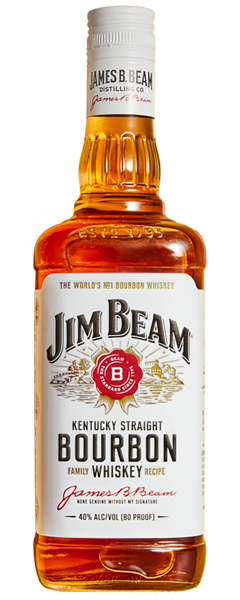The image features a bottle of Jim Beam bourbon whiskey set against a white or transparent background. The bottle is made of glass and contains an amber-colored liquid, indicating the whiskey inside. It is topped with a distinctive white lid.

The label of the bottle is predominantly white and provides detailed information about the product. At the top of the label, "James B. Beam Distilling Company" is prominently displayed along with what appears to be a signature, presumably of James B. Beam. The main part of the label reads "The World's No. 1 Bourbon Whiskey" or something similar, emphasizing its renowned status. The central portion features the brand name "Jim Beam" accompanied by a prominent "B" emblem reminiscent of a prize-winning medallion.

Below, the label elaborates "Kentucky Straight Bourbon Family Whiskey Recipe" followed by "James B. Beam". Some additional, finer text is present but is too small to be legible in the image. Lastly, the label states the alcohol content of 40% (80 proof), reiterating that this is a bottle of Jim Beam bourbon whiskey.